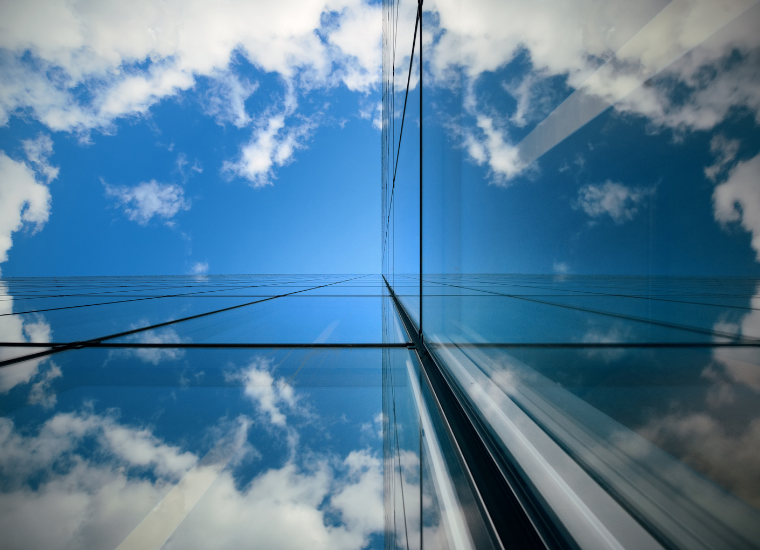The image captures an upward view from the corner of a glass-faced skyscraper, highlighting the striking reflection of the bright blue sky and scattered white clouds on the building's reflective surface. The photo, taken from the ground level at a 90-degree angle, creates an almost seamless visual merge between the sky and its mirrored reflection on the glass panels. The clear, color photograph boasts vivid details, emphasizing the expansive, cloud-dotted sky that appears to slice through the image, with the reflective building seemingly extending infinitely upwards. The right-hand edge of the photo features a subtle contrast with some white and black hues but remains dominated by the reflective glass and the stunning sky. The overall setting is bright and well-lit, offering a crisp and clear view that leaves the sky and its reflection as the primary focus.